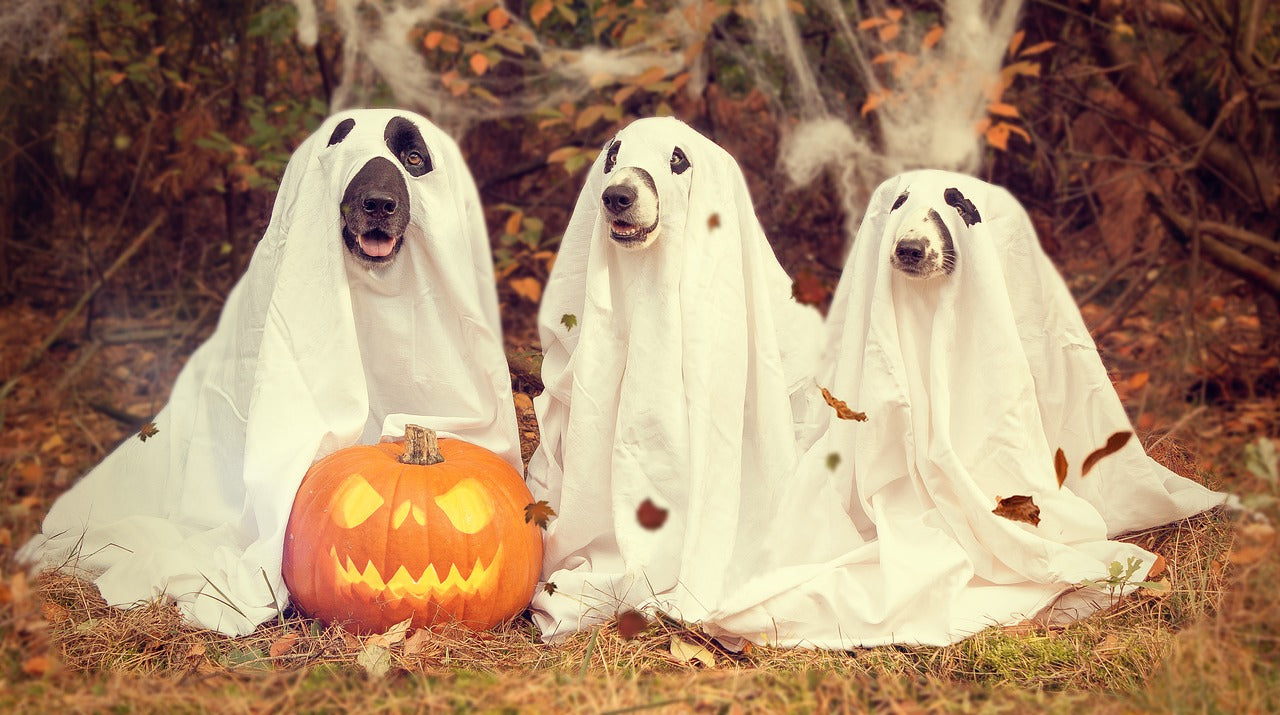In this detailed outdoor daytime photograph taken during fall, three medium-sized dogs sit side by side, dressed in white sheets with holes cut out for their eyes and snouts, resembling ghosts. The dog on the left has a black face and sits in front of an orange jack-o-lantern with a carved, illuminated skeleton face. The two dogs on the right each have white snouts with black around their eyes and, like the dog on the left, sport black noses. The scene is set on a patch of yellowish-green grass, surrounded by brownish leaves and trees. In the background, we see cotton-like fake spiderwebs randomly placed among the trees, enhancing the spooky Halloween ambiance. The vivid colors in the image include shades of orange, brown, yellow, white, pink, light orange, light brown, and black, adding to the seasonal setting.